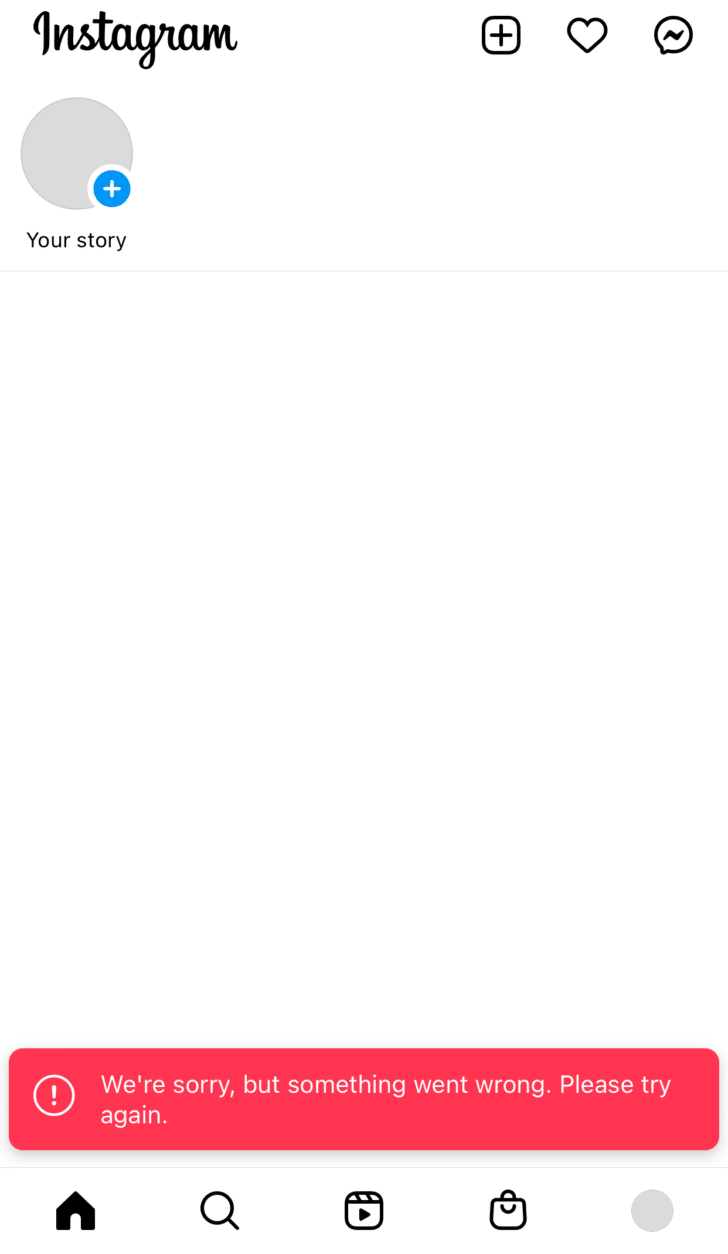This image appears to be a screenshot taken from a social media app, specifically Instagram, viewed on a phone or tablet. At the top, the traditional cursive "Instagram" logo is displayed. To the right of the logo, there are three icons: a square with a plus sign, a heart, and a message bubble with what appears to be a lightning bolt highlight. 

The overall image has a white background with no visible borders on the sides. Below the "Instagram" logo, there is a gray circle and a blue circle with a plus sign, labeled "Your Story." A thin gray line separates this section from the next.

In the main content area, a red rectangular button is prominent, accompanied by a circle with an exclamation mark, displaying the message, "We're sorry, but something went wrong. Please try again." A thin line further separates this section from the bottom navigation bar.

The bottom navigation bar includes a house icon, which is highlighted in black, a magnifying glass icon, a play button icon likely meant for media, a purse icon probably indicating shopping, and a gray circle.